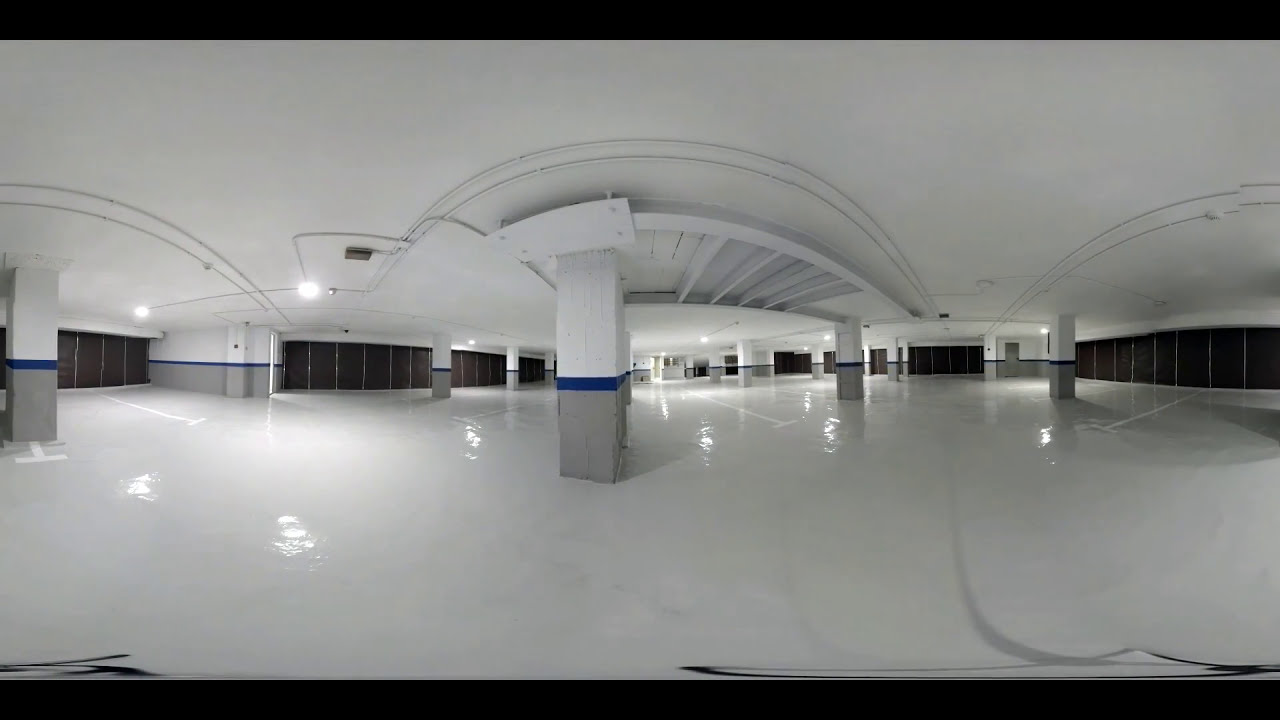The image depicts the interior of what appears to be an empty, high-end parking garage. The smooth, shiny floor is exceptionally clean, giving off a slightly reflective, almost icy appearance. The large space is supported by several sturdy pillars, each distinguished by their three-tone coloration: a gray base, followed by a blue stripe, and then topped with white stretching up to the ceiling. The walls mirror this design, maintaining the same color scheme. The ceiling itself is designed with a slight curve and holds lights that illuminate the entire area. White parking markings line the floor, organized neatly for parking stalls. In the distance, windows and doorways are visible, hinting at more spaces or potential exits. No cars, people, or text are present in the image, adding to the clean and untouched atmosphere of the garage. The overall photo has a slight warping effect around the edges, suggesting it might be taken from a security camera or have some VR-like distortion.